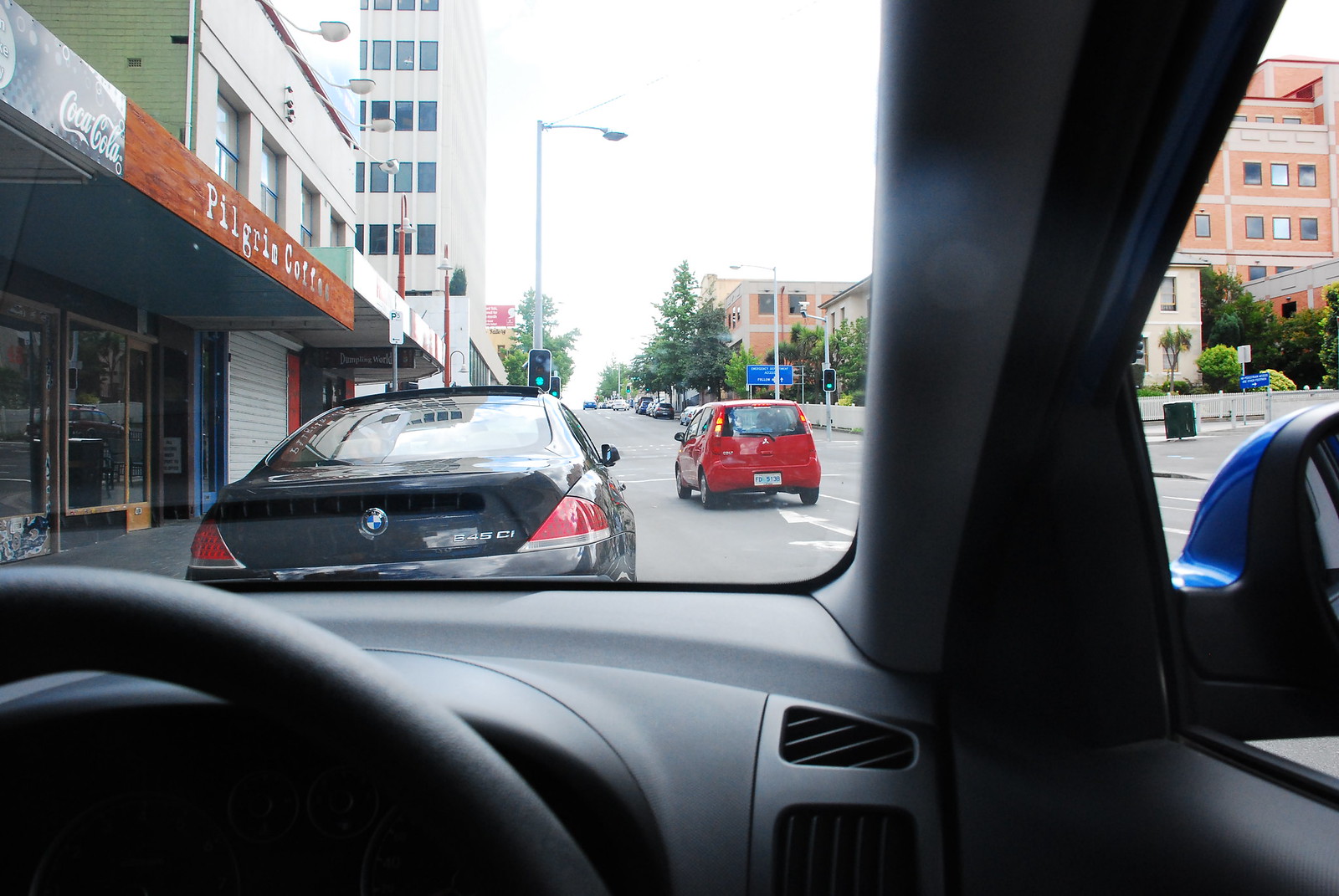The interior of the PAR includes a plastic dashboard with air vents positioned to the right side. At the forefront, there is a steering wheel encased in a plastic trim. The view through the right window reveals a detailed urban scene. A large red building with black windows dominates the far right side. 

On the road, a red car is seen driving forward. To the left of the red car, a BMW is parked. Further left, there is another building that either appears to be a pizzeria or a café named "Pilgrim Coffee." 

This building prominently features a Coca-Cola sign in black with white cursive lettering. Behind these foreground elements, a large white building stands amidst a backdrop of green trees against a white sky.